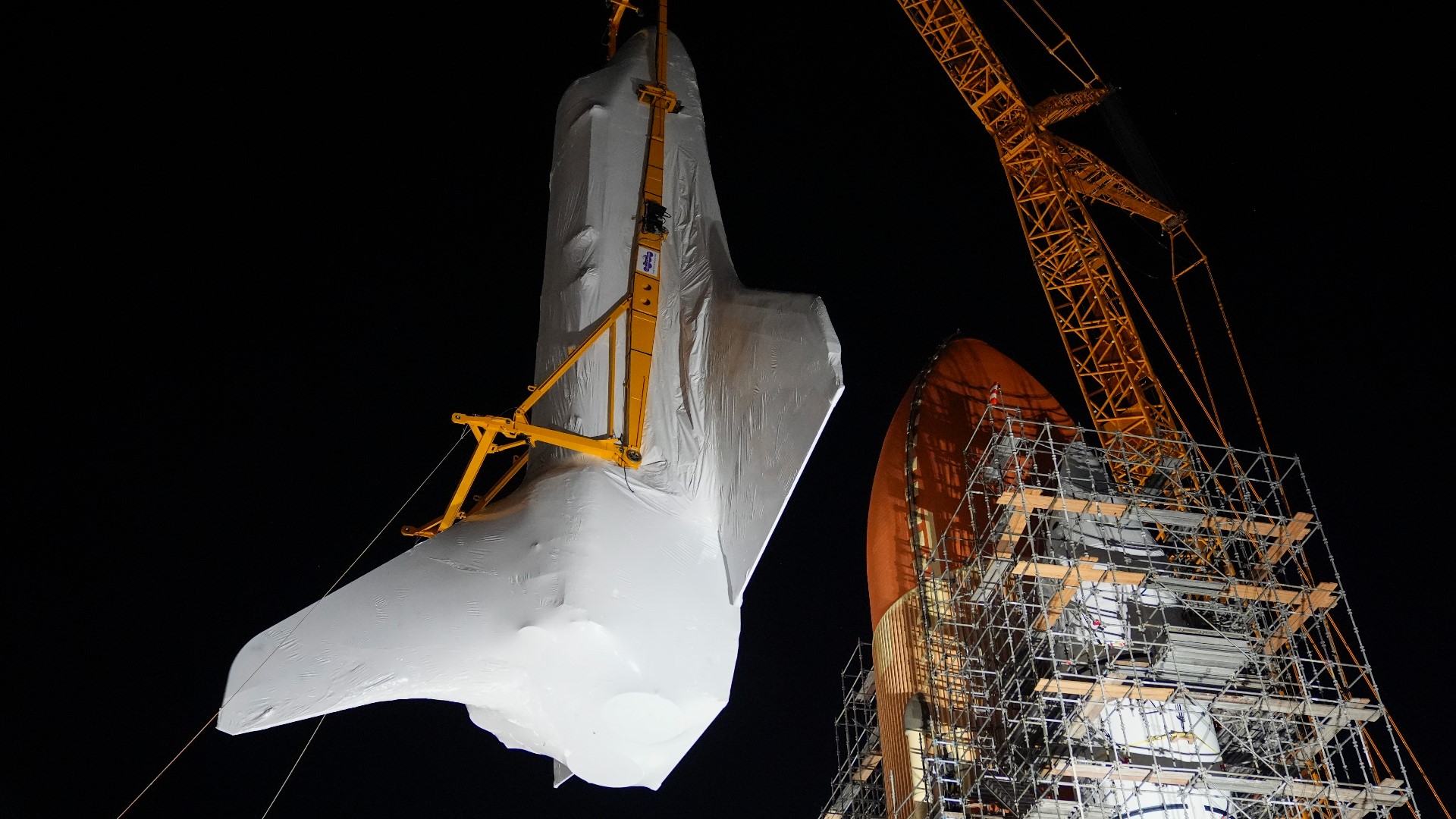This nighttime photograph captures a dramatic scene at what appears to be a NASA facility or the California Science Museum. The background is completely pitch black, highlighting the industrial and high-tech elements of the setting. Dominating the right-hand side of the image is an immense, towering orange crane, stretching stories high into the night sky. The crane is in the process of hoisting a space shuttle orbiter, which is meticulously wrapped in a protective white cloak. The boosters of the shuttle are visible, protruding from the bottom of the covering. To the left of the crane, there is a massive tubular object, likely an external tank, surrounded by gray scaffolding and rigging, ready to be connected to the shuttle. Orange arms are attached to both the shuttle and the tank, possibly serving as guide wires. A subtle light source, possibly a spotlight, illuminates the scene from below, adding a dramatic effect to the meticulous nighttime operation. The image beautifully encapsulates the scale and complexity of space exploration technology.